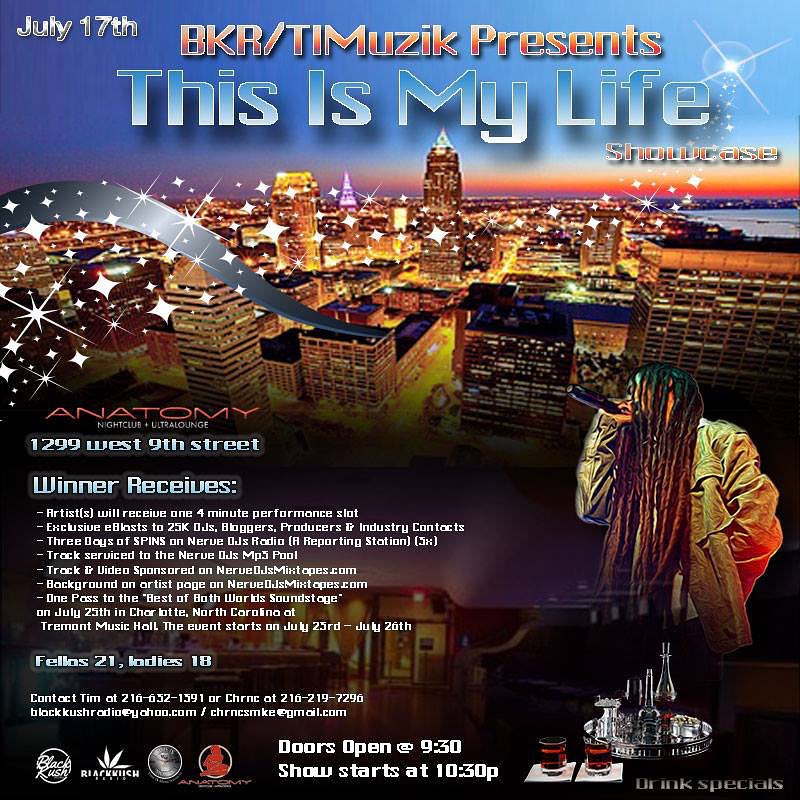The image is an advertisement for a music showcase event named "This is My Life Showcase," presented by BKR/TI Music on July 17th. The backdrop features a lit-up cityscape, suggesting a vibrant urban setting. At the top left corner, the date "July 17th" is prominently displayed. The event will be held at Anatomy Nightclub and Ultra Lounge, located at 1299 West 9th Street. 

On the right side of the image, there's a performer with long dreadlocks, his face obscured by his hair, holding a microphone, suggesting a live performance aspect. Additionally, there is an image of a drinks tray with bottles and glasses indicating drink specials available at the event. 

The ad mentions several details about the event: winners of the showcase will receive a 4-minute performance slot, an exclusive e-blast sent to 25,000 DJs, bloggers, producers, and industry contacts, and three days of spins on Nerve DJs Radio, a reporting station. Entry requirements state that men must be 21 years or older and women 18 years or older. Doors open at 9:30 PM, with the show starting at 10:30 PM.